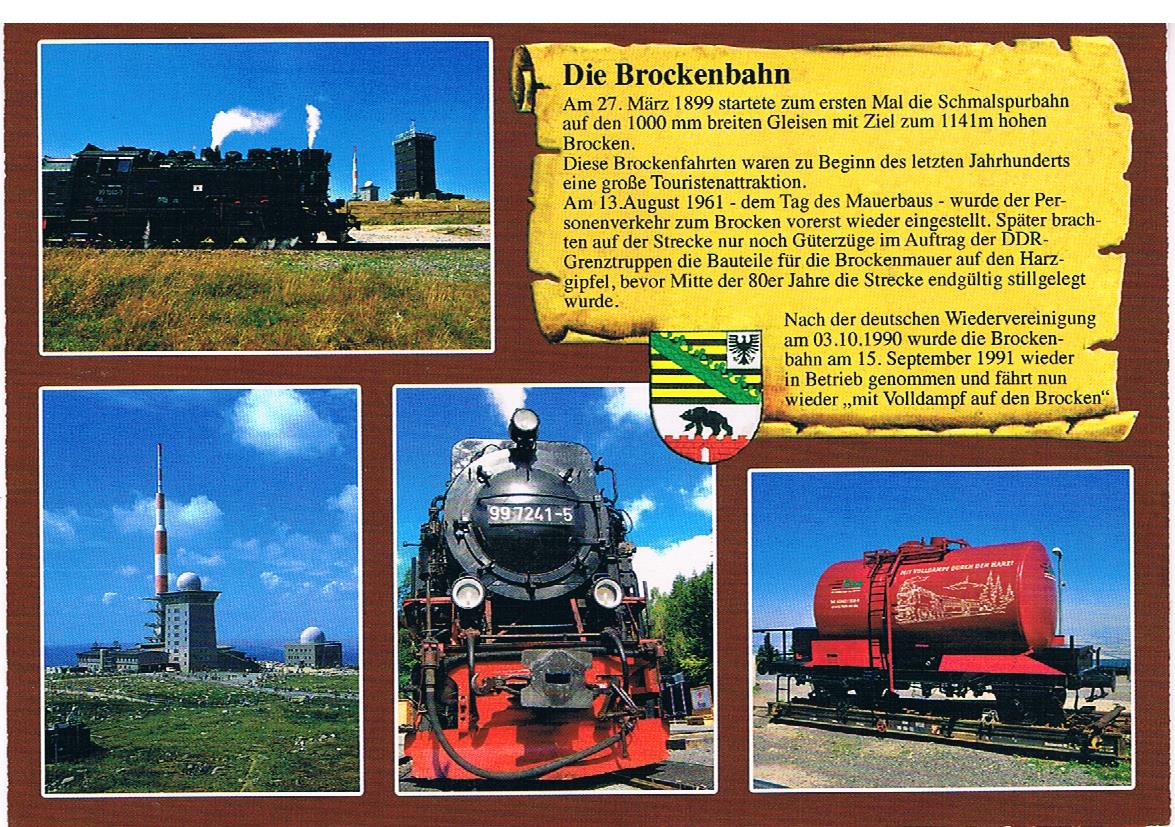This photograph showcases a detailed flyer or advertisement for the Brockenbahn train, set against a dark brown background. The flyer is sectioned into four images, along with a prominent yellow scroll-like graphic and a distinctive crest.

In the top left image, we see a striking black steam locomotive moving across a grassy foreground under a clear blue sky, with white smoke billowing from its chimney. The bottom left photo features a complex structure that includes a large gray building with a white dome, and a smaller similar building to its right, accompanied by a red and white striped pole. The adjacent bottom center photograph presents a close-up of the locomotive's front, prominently displaying the number 997-241-5 and featuring a striking red lower front. The bottom right image captures the train's vibrant red caboose against a backdrop of blue sky, highlighting the ladder along its side and the rocky terrain beneath.

To the top right of the bottom center photo is an intricate crest, depicting a bear-like animal traversing a red rock ledge with yellow and black stripes above, a green sash diagonally crossing from upper left to lower right, and a bird or eagle positioned in the top right corner. Adjacent to this crest, nestled in the flyer’s upper right corner, is the eye-catching yellow scroll. This scroll, adorned with text in an elegant Times New Roman font, is inscribed in German, reading "Die Brockenbahn" with the date "AM 27 März 1899." Though the specific German text is unreadable to a non-German speaker, it adds an authentic, historical touch to the overall design.